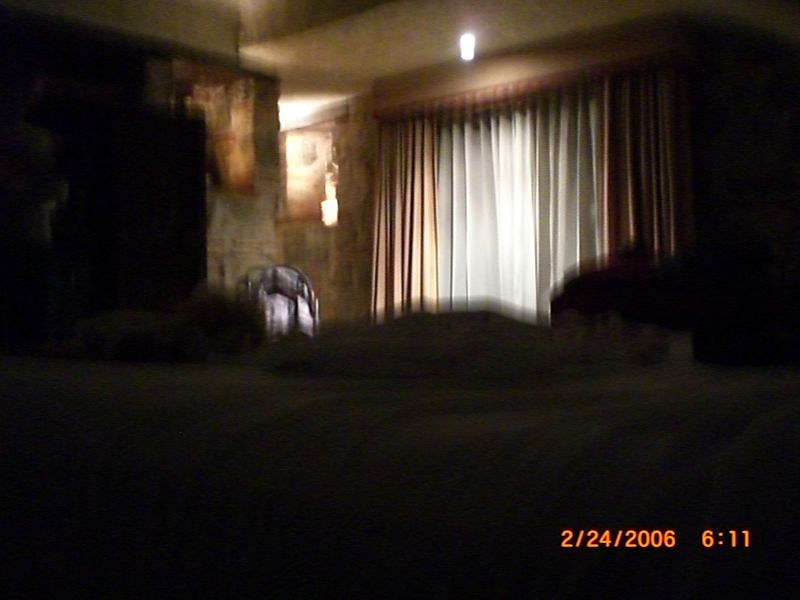A blurry, low-quality image captures a cozy bedroom from an unusual side angle, as if taken from the head of the bed near the headrest. In the foreground, you can see the neatly made bed with visible sheets. The background reveals a charming brick wall and a sliding door covered by rich, reddish curtains with a white underlay, giving the room a slightly darkened and warm atmosphere.